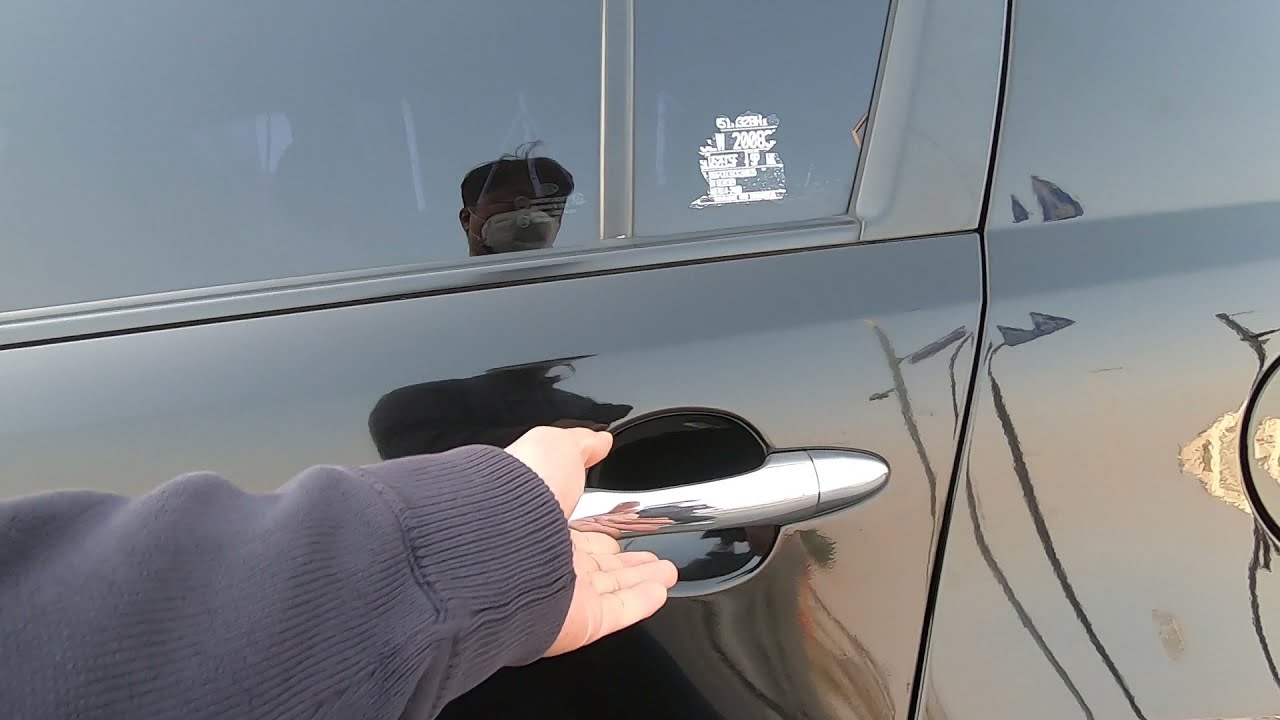The photograph captures a close-up view of a shiny black car door with a silver handle. An arm clad in a gray sweatshirt or sweater, extending from the elbow, is reaching for the handle. The hand is light-skinned, suggesting the person is likely caucasian, and appears to be poised to open the door. Reflected on the car's window is the image of a man with short dark hair wearing a white surgical mask. Additionally, the window features a small white sticker or decal partially visible in the corner, with some illegible text and the number "2000." Various reflections, including those of streetlights and possibly street signs, can also be seen on the car's glossy surface.